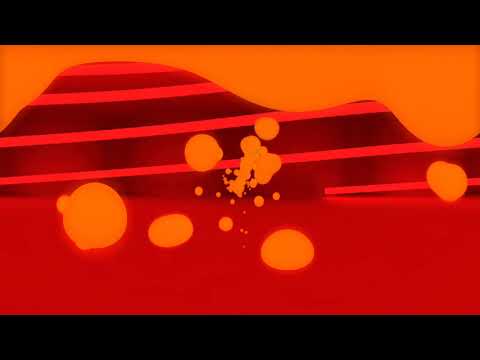The image is a vibrant screenshot, possibly from a movie or cartoon, characterized by a dynamic array of reds, oranges, and dark hues. Dominating the scene is an evocative composition reminiscent of molten metal or a lava lamp, with a dramatic interplay of orange bubbles or blobs of various sizes hovering and drifting towards a larger central blob. These abstract shapes, appearing in a striking orangish hue, float amidst a dark red backdrop adorned with bright red diagonal stripes. The foreground features a flat, dark red expanse, while the background hosts a dark red gradient with prominent orange stripes. Intense orange sky and curved mountain silhouettes span horizontally across the image, painted with bright red stripes, adding a sense of surreal landscape against two black bars that frame the top and bottom of the image.